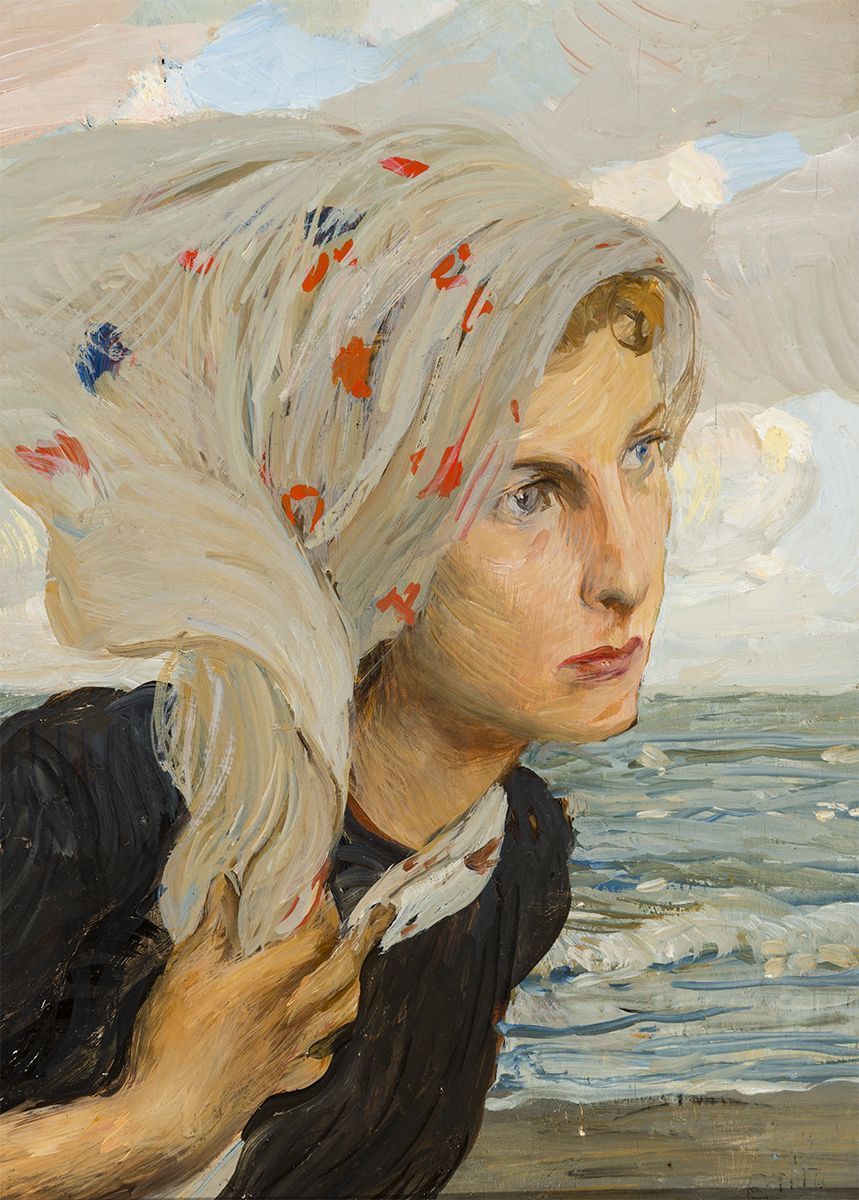The oil painting depicts a Caucasian woman in her mid-30s to 40s standing on a beach under a cloudy sky. Her blonde or auburn hair peeks out from beneath a white scarf, which she is holding tight around her head with her right hand. The scarf is adorned with dots of red, orange, and blue, and its texture is rendered with creamy, stringy brush strokes. She has fair skin, blue or bluish-hazel eyes, and wears red lipstick. Her outfit consists of a dark-colored, short-sleeved shirt, possibly black or gray. The woman is shown from her bust up, leaning slightly forward and gazing into the distance with a thoughtful expression. In the background, the ocean's waves are painted with bold strokes of blue, gray, and white, meeting the beige-brown sandy shore. The overall effect is soft and detailed, capturing both the serene and dynamic elements of the scene.